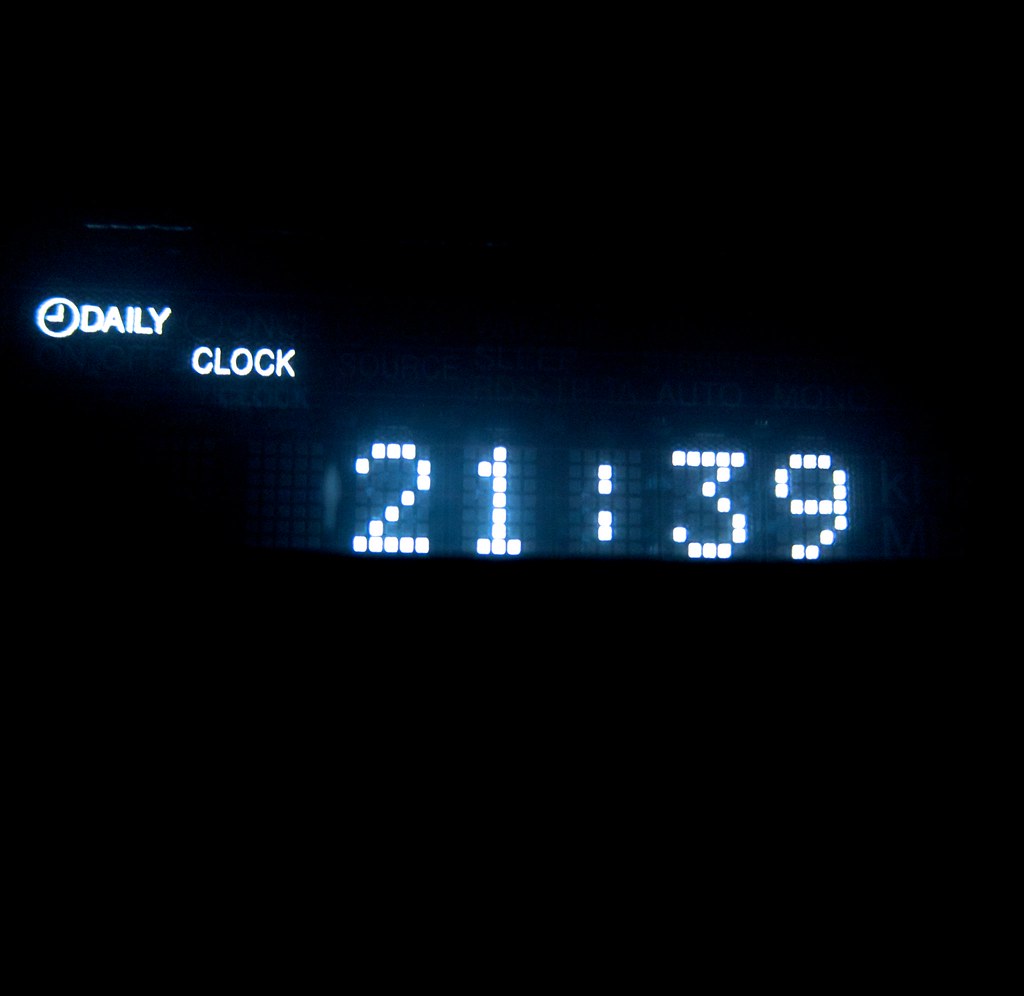This image depicts an illuminated digital clock display against a pitch-black background, with no visible outline of the clock itself. The clock reads "21:39" in large, white numerals formed by small, glowing cubes. Positioned in the upper left corner, an analog clock image showing 9 p.m. is accompanied by the word "DAILY" in capital letters. Below and slightly to the right, the word "CLOCK" is displayed in smaller text. Additional, less prominent text includes labels like "on/off", "source", "ROD 3", "auto", "mono", and "select," arranged around the main display area. This setup suggests a digital alarm clock configured to a 24-hour format, indicating a set daily alarm.